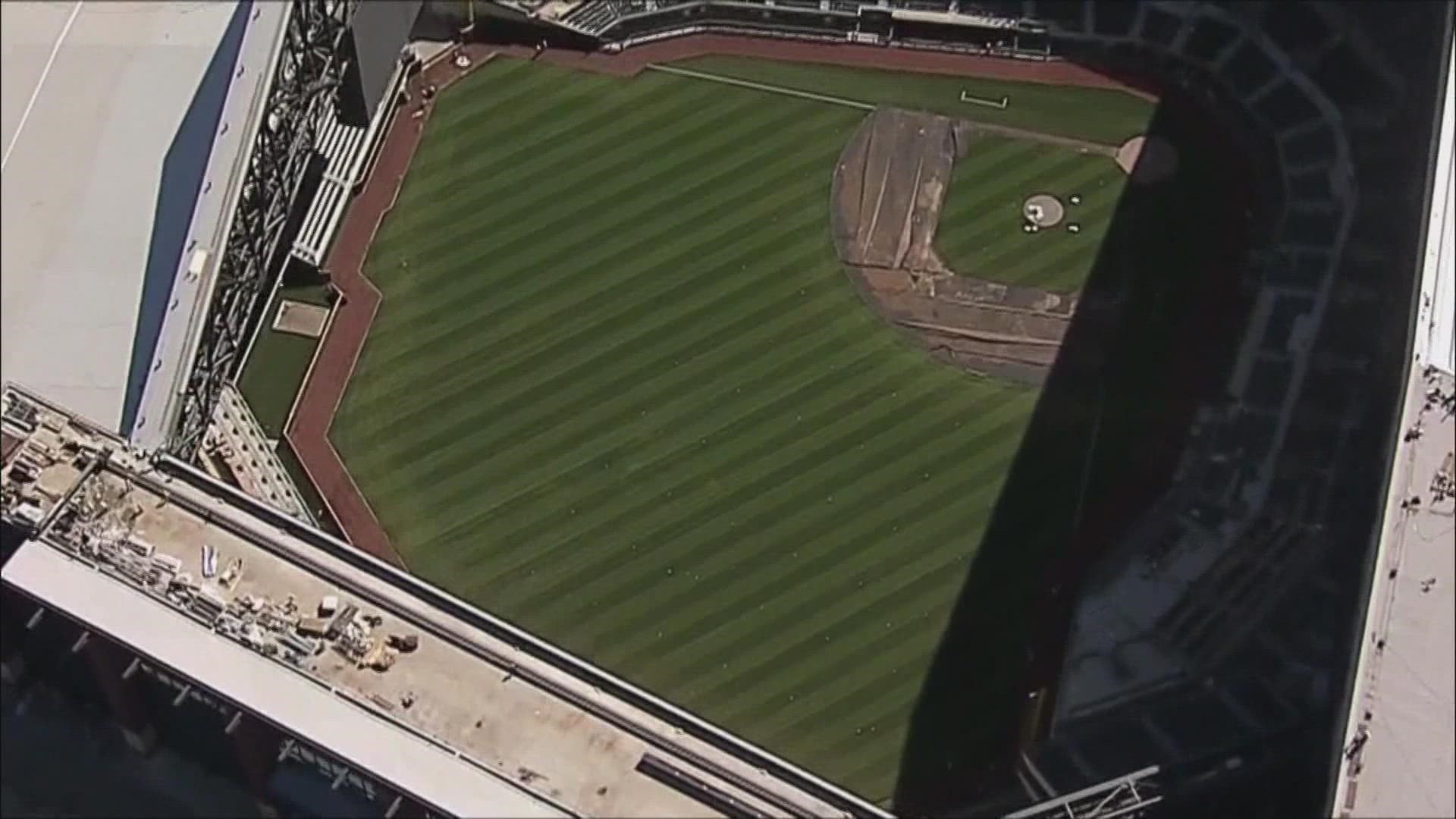The image captures an aerial perspective of a baseball stadium on a partly cloudy day, showing a stark contrast between sunlight and shadows. The stadium has distinctive diagonal cuts in the grass, alternating between light and dark green. The baseball diamond is clearly visible at the center, with home plate and the batter’s box located near the deeply shadowed portion of the field, which suggests the heavy shadows cast by extensive, tiered bleachers or walls on the right-hand side. The stands appear empty and are shrouded in darkness, hinting at the possibility of it being early morning or late afternoon.

In the foreground, the bottom left of the image reveals part of the stadium's infrastructure, including a light-colored, likely gray, roof with visible trusses and an adjacent area that seems to be under construction, cluttered with white boxes and equipment. The image quality seems slightly overcast, adding a greyish tone overall, reminiscent of a low-quality screenshot possibly taken from a news helicopter flyover. The view doesn't encompass the entire stadium but offers a detailed glimpse of the field's layout, the surrounding architecture, and the stark division between sunlight and shadow.